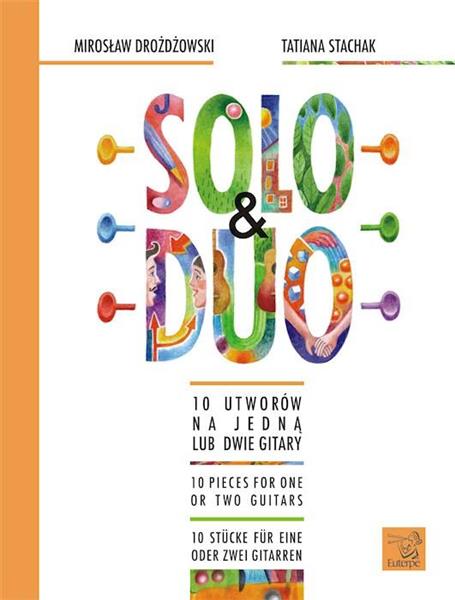This vibrant poster, which resembles the front cover of a book or magazine, prominently features an orange bar along the left edge and an orange square with an icon in the bottom right corner. At the top, the names Miroslav Drodzewski and Tatiana Stachak are displayed in black text on the left and right respectively. The centerpiece of the poster is a large, colorful, block capital text that reads "Solo and Duo," with the ampersand symbol in black. Beneath this, it is subtitled with "Ten pieces for one or two guitars" in English, accompanied by additional text in another language. The poster uses a vibrant palette including white, orange, black, pink, purple, blue, green, and brown, effectively capturing attention with its artistic design and diverse colors. The structured layout and vivid hues suggest it may be advertising a concert or similar event.